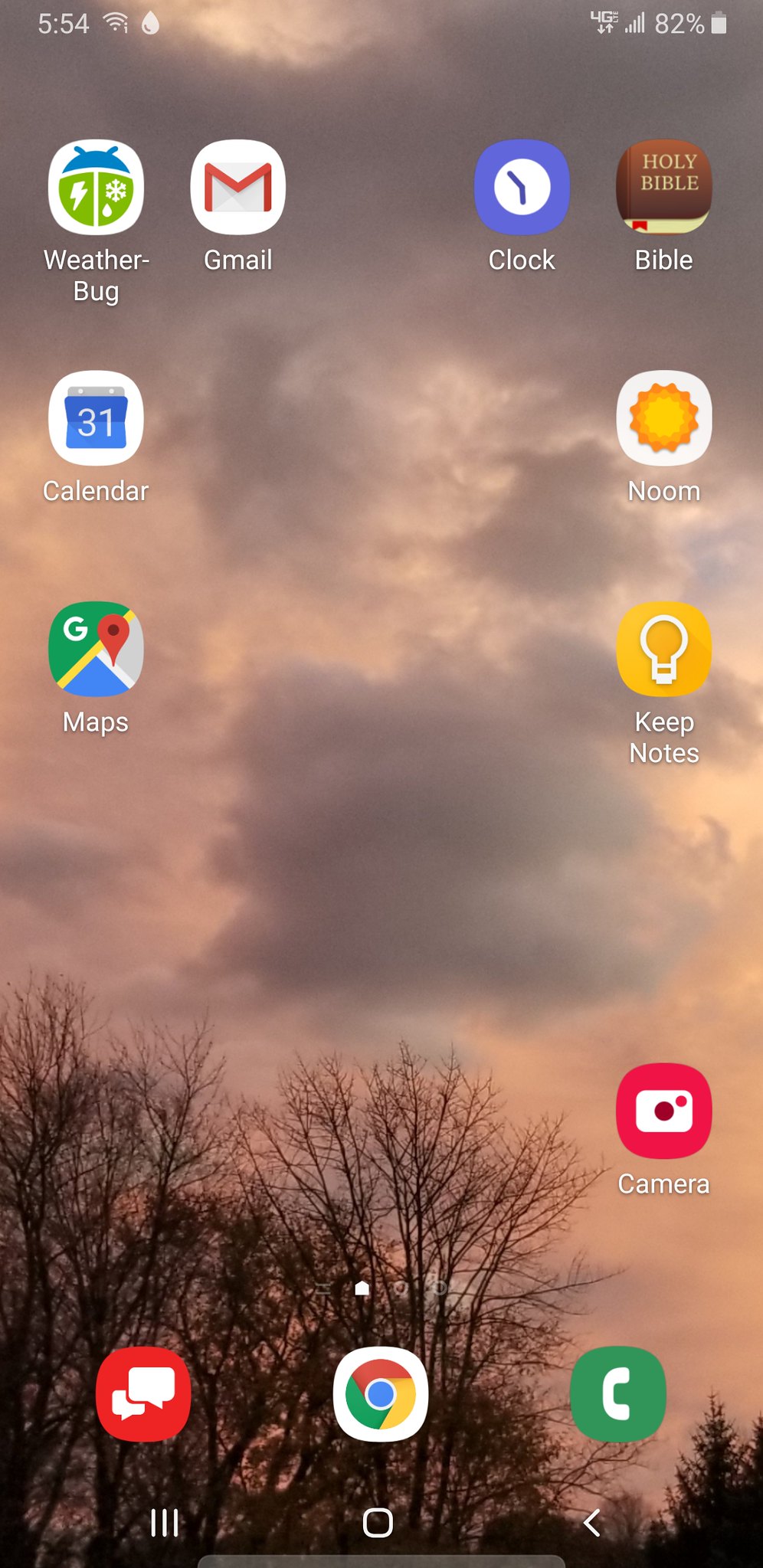The home screen of a smartphone displays various app icons against a backdrop of bare trees and cloudy sky. The status bar at the top shows the time as 5:54, with full mobile signal represented by five ascending bars, 4G internet connectivity, and an 82% battery level indicated by a mostly filled white battery icon. 

On the home screen, the top row features the WeatherBug app, identifiable by its blue bug icon with green lightning and weather symbols, followed by the Gmail app, and a clock app displaying clock hands. The Holy Bible app with a brown cover and gold cross is also present.

The next row includes the Calendar app and a noon app, slightly separated from each other. The Maps app is on the left side, while the Keep Notes app is positioned on the right.

Towards the bottom of the screen, there's a Camera app followed by a gap, then a series of apps including a red Text Messaging app, Google Chrome, and WhatsApp, which is distinguished by a green icon with a white phone symbol.

Overall, the screen composition is neatly organized with a serene background image of leafless trees and a cloudy sky providing a calm yet wintry atmosphere.